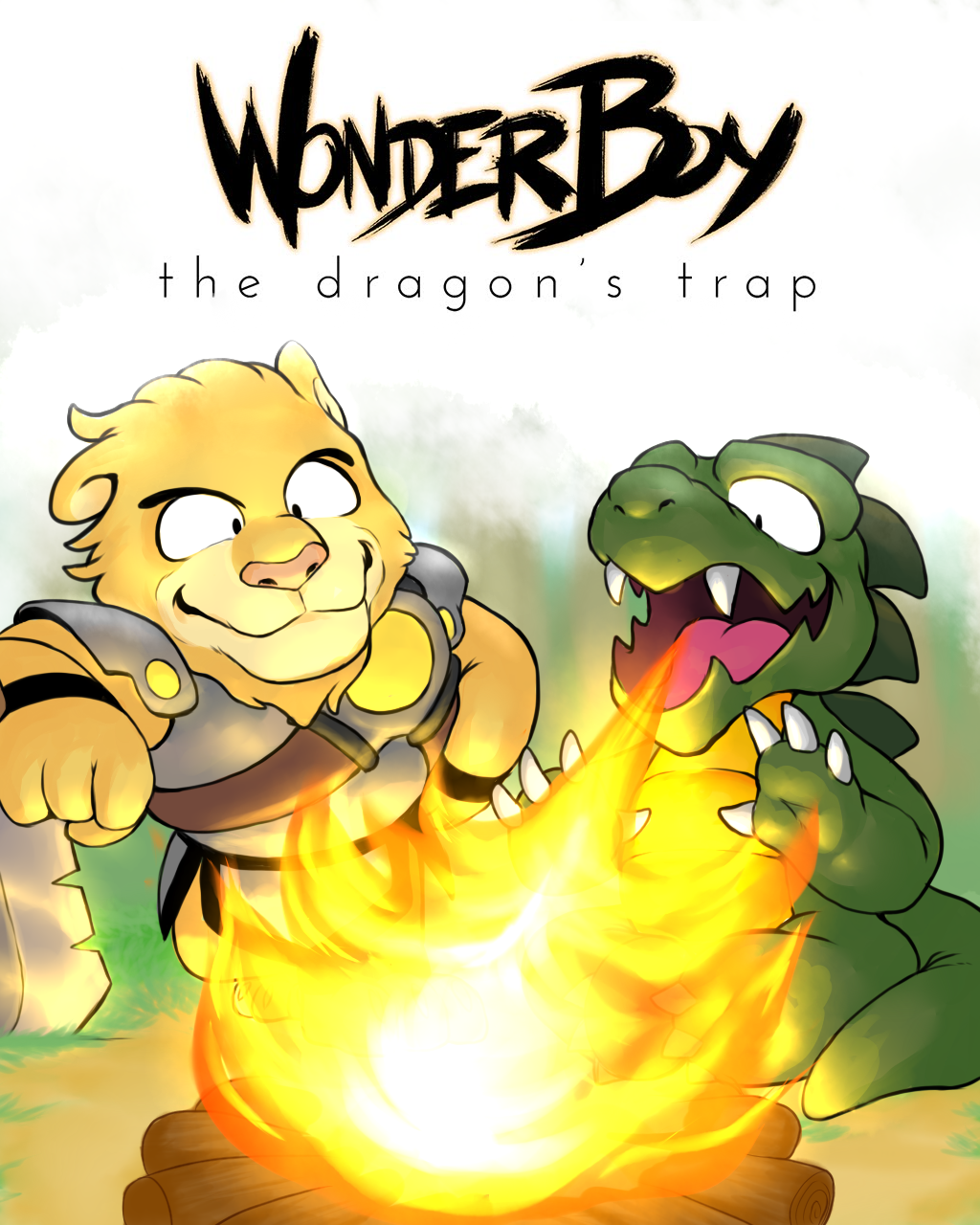The artwork showcases a promotional piece for the game "Wonder Boy, the Dragon's Trap," with the title prominently displayed at the top. "Wonder Boy" appears in bold, black calligraphy with a golden border, while "the Dragon's Trap" is written in lowercase letters below it. Below the title, two anthropomorphic creatures are depicted. To the left is a yellow lion with a pink nose, clad in silver and brown plate armor, accented by black armbands and a belt with a large yellow stone on the buckle extending from his left shoulder. The lion is leaning on a pitted sword. To the right is a green, dinosaur-like dragon with a gold belly, breathing fire towards the middle of the image. The flames are vividly colored in yellow, orange, and white, suggesting they are gathered around a campfire. The background has a hazy green and white theme, contributing to the image's cartoonish and Japanese anime feel. The detailed and expressive art style enhances the fantastical elements of the scene.